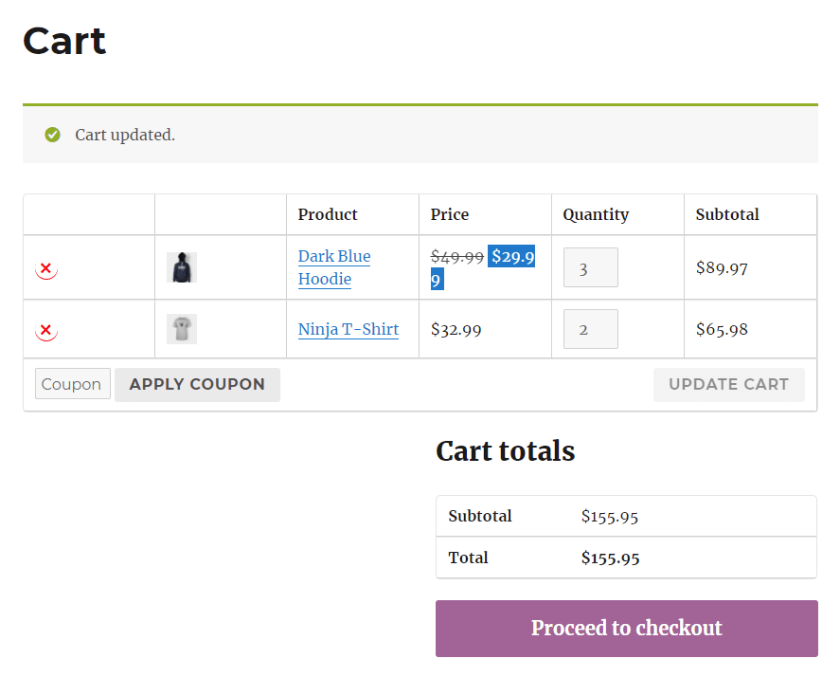**Screenshot of Online Shopping Cart**

At the top of the screenshot, the page title reads "Cart," accompanied by a thin horizontal green line. Beneath that, a notification in green text states "Cart Updated," adjacent to a green circle with a white check mark inside of it.

The cart displays two items:

1. **Product**: Dark Blue Hoodie
   - **Original Price**: $49.99 (crossed out)
   - **Discounted Price**: $29.99
   - **Quantity**: 3
   - **Subtotal**: $89.97

2. **Product**: Ninja T-Shirt (Gray)
   - **Price**: $32.99
   - **Quantity**: 2
   - **Subtotal**: $65.98

Further down, there are options to apply a coupon and update the cart, followed by the cart totals:

- **Subtotal**: $155.95
- **Total**: $155.95

At the bottom, a call-to-action button reads "Proceed to Checkout" in white text, set within a purple rectangle.

The screenshot does not include any images of people, animals, plants, flowers, or trees.